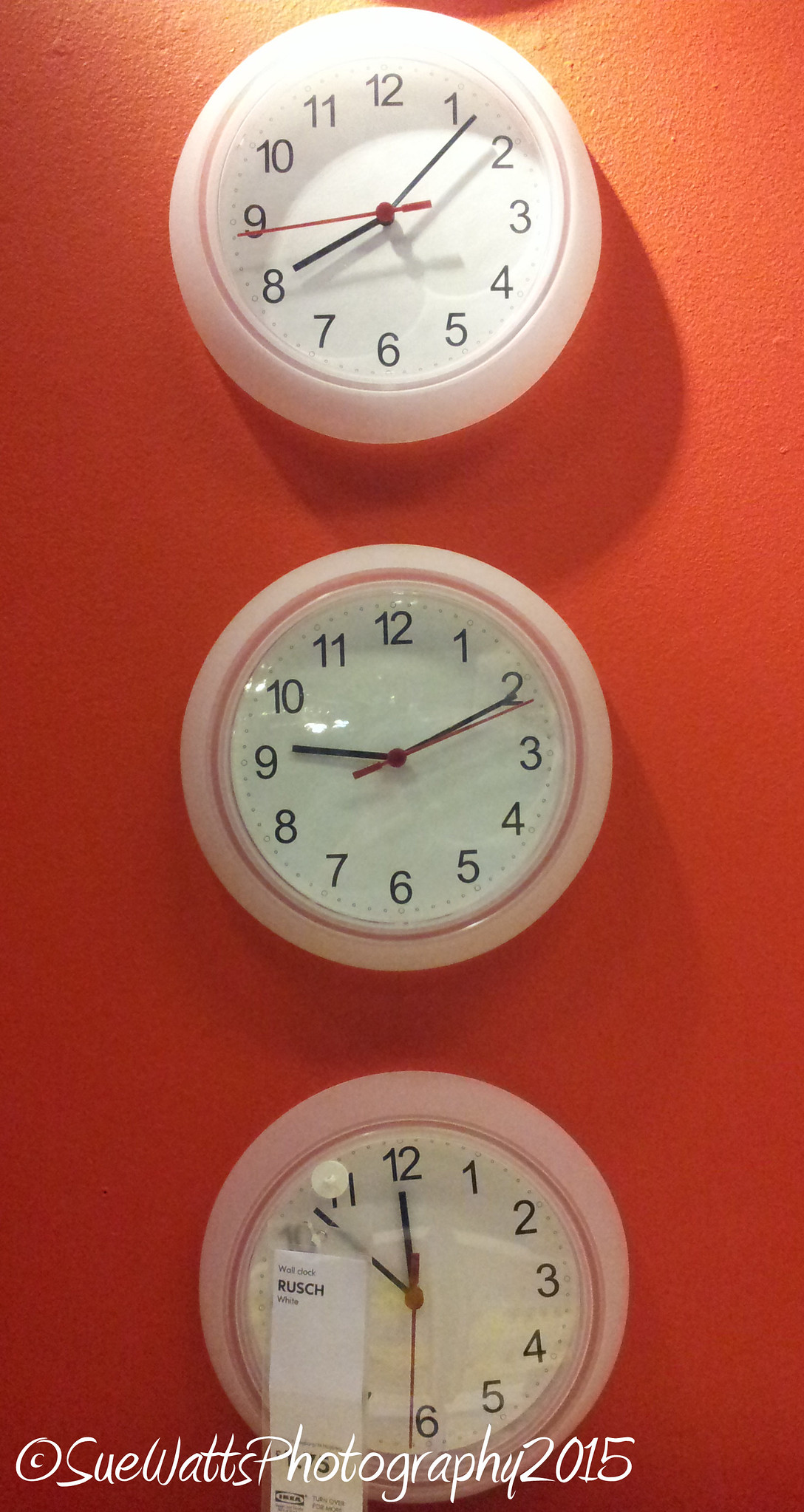Photographed by Sioux Watts Photography in 2015, this striking image showcases three distinct clocks against a vibrant gradient backdrop that transitions from deep red at the bottom to bright yellow at the top. The first clock, positioned on the left, appears devoid of a glass cover, revealing its clean white face with black hour and minute hands and a contrasting red second hand. Its rim is subtly pink, though it's not immediately apparent. The second clock, identical in design to the first, features a clearly visible glass cover with reflective highlights. It also has a pink rim that is slightly more evident than the first. The third clock, also protected by a glass cover, is distinctively marked by a white tag taped near the 11 o'clock position. The tag prominently displays the word "BUSCH" in bold letters, followed by additional text in a vertical arrangement. All three clocks are set against the richly colored background, creating a visually dynamic and detailed composition.